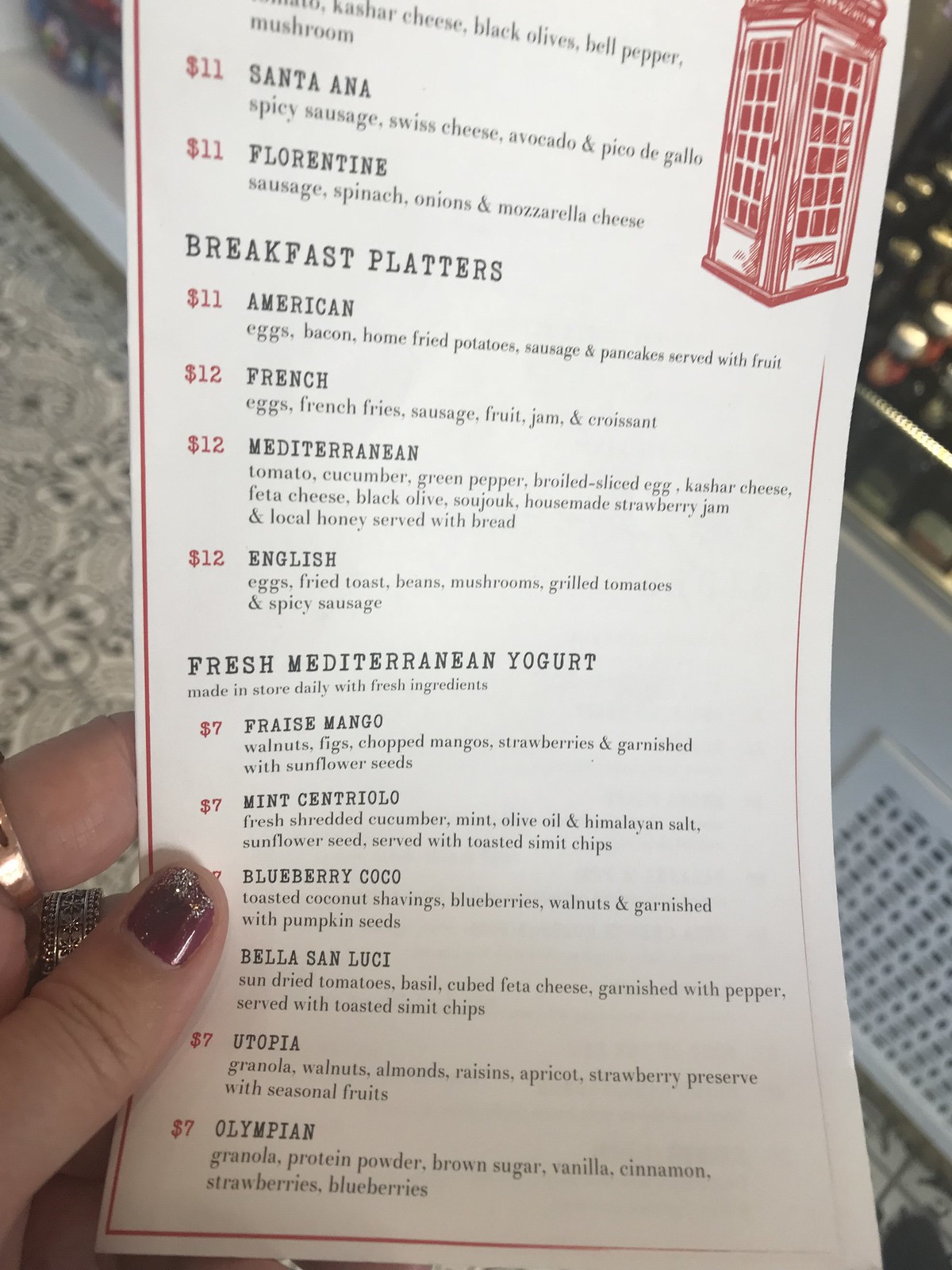In the image, a menu for a breakfast restaurant is prominently displayed. The menu features a variety of Spanish-inspired dishes, suggesting an authentic Spanish theme, rather than a broader Latin American influence. The specific items and categories listed include:

1. **Santa Ana:** Spicy sausage, Swiss cheese, avocado, and pico de gallo.
2. **Florentine:** Sausage, spinach, onions, and mozzarella cheese.
3. **Breakfast Platters:**
   - **American Platter:** Eggs, bacon, home-fried potatoes, sausage, and pancakes served with fruit.
   - **Mediterranean Breakfast Platter:** Tomato, cucumber, green pepper, broiled sliced egg, kasha cheese, feta cheese, black olive, sujuk, house-made strawberry jam, and local honey served with bread.

Additionally, there is a category for "Fresh Mediterranean Yogurt." 

In the upper right corner of the menu, a red and white illustration depicts what appears to be a small room or cell-like structure, with a door featuring a caged pattern and glass, reminiscent of a time machine’s depiction in popular media.

A woman's hand, adorned with red nail polish and a ring, holds the menu, adding a human element to the scene.